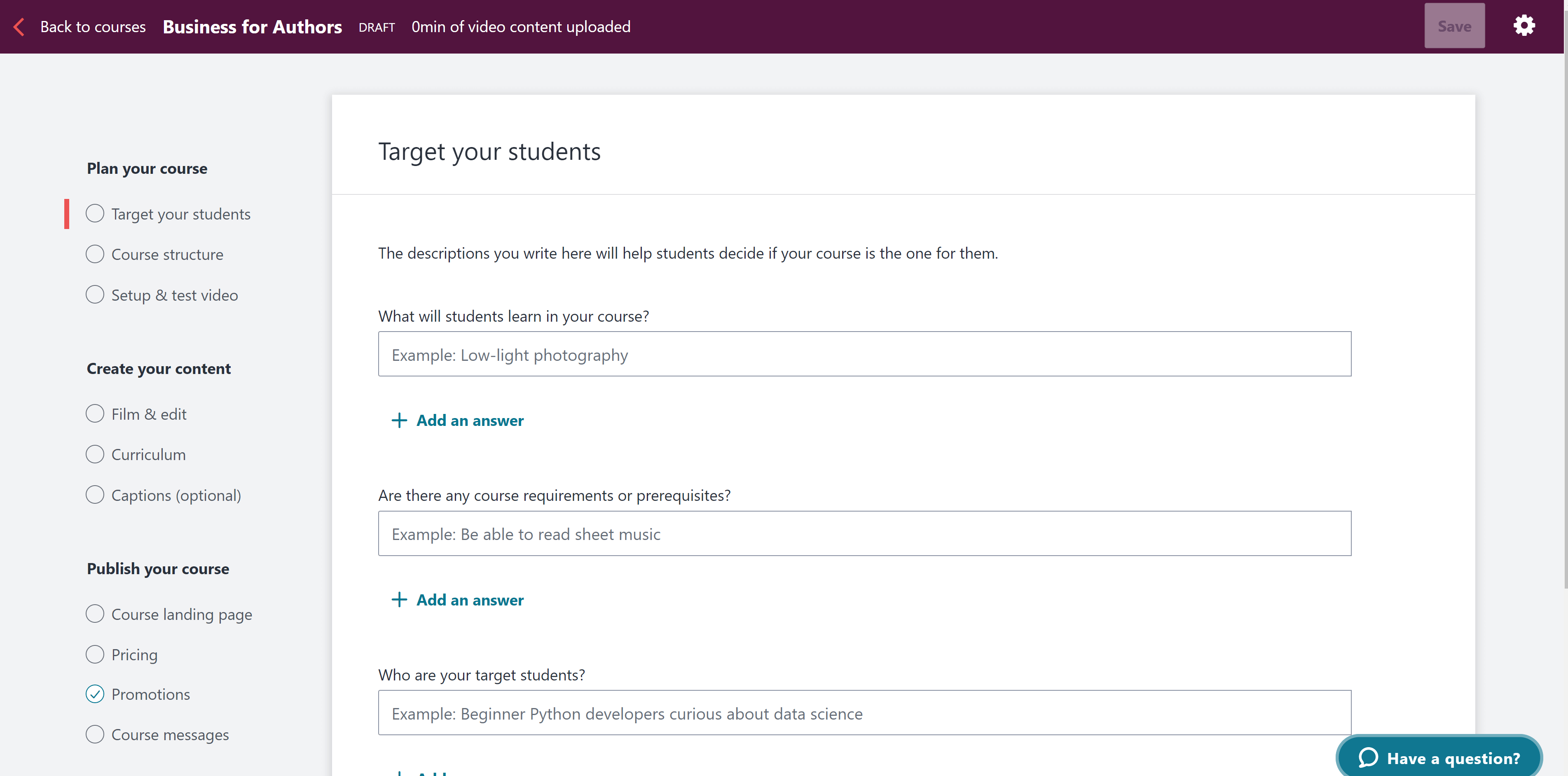This screenshot showcases a section within an application or web interface titled "Business for Authors." At the top, there is a burgundy-colored banner with a back arrow labeled "Back to Courses." Clicking this arrow navigates you back to the main courses section. Centered in bold, larger text is the title "Business for Authors," followed by the word "Draft" and the note "0 minutes of video content uploaded" in unbolded text. On the far right of the banner, there is a gray "Save" button alongside a gear icon for accessing settings.

The main interface is divided into two sections. On the left, a column allows you to navigate through different course creation stages: "Plan Your Course," "Create Your Content," and "Publish Your Course." Each stage lists three or four specific tasks with selection bubbles beside them. The current selection, indicated by a green check mark, is "Promotions" under the "Publish Your Course" section.

On the right, the interface includes several form fields under the heading "Target Your Students: The decisions you make here will help students decide if your course is the one for them." The form asks for information about what students will learn in the course, any course requirements or prerequisites, and who the target students are. Each query has a corresponding text box for the user to fill in.

In the bottom right-hand corner, there is a blue button with a speech bubble icon labeled "Have a Question," which initiates a chatbot for further assistance.